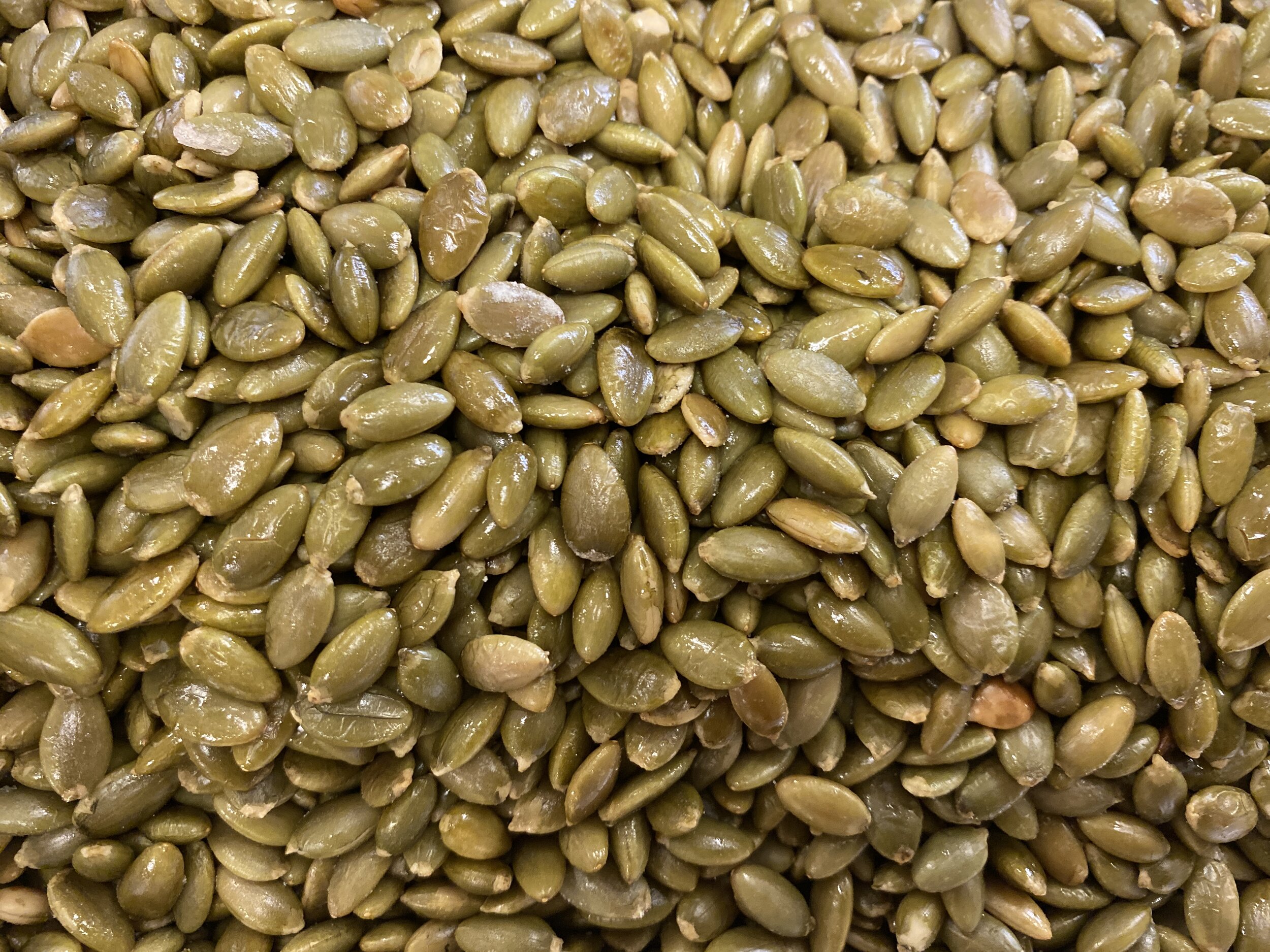The image showcases a vast pile of what appears to be pumpkin seeds, also known as pepitas, completely filling the frame from edge to edge. These seeds, devoid of their outer shells, display a variety of colors, including different shades of green, olive, yellowish, and brown. Their shiny, possibly oily surface glistens under the light, suggesting a slick or slimy texture. Some seeds also seem to have grains of salt sprinkled on them, adding to their diverse texture. This dense, uncountable mass of seeds, in myriad hues, creates an intricate tapestry of color and texture, capturing the complexity and beauty of these simple yet varied pumpkin seeds.